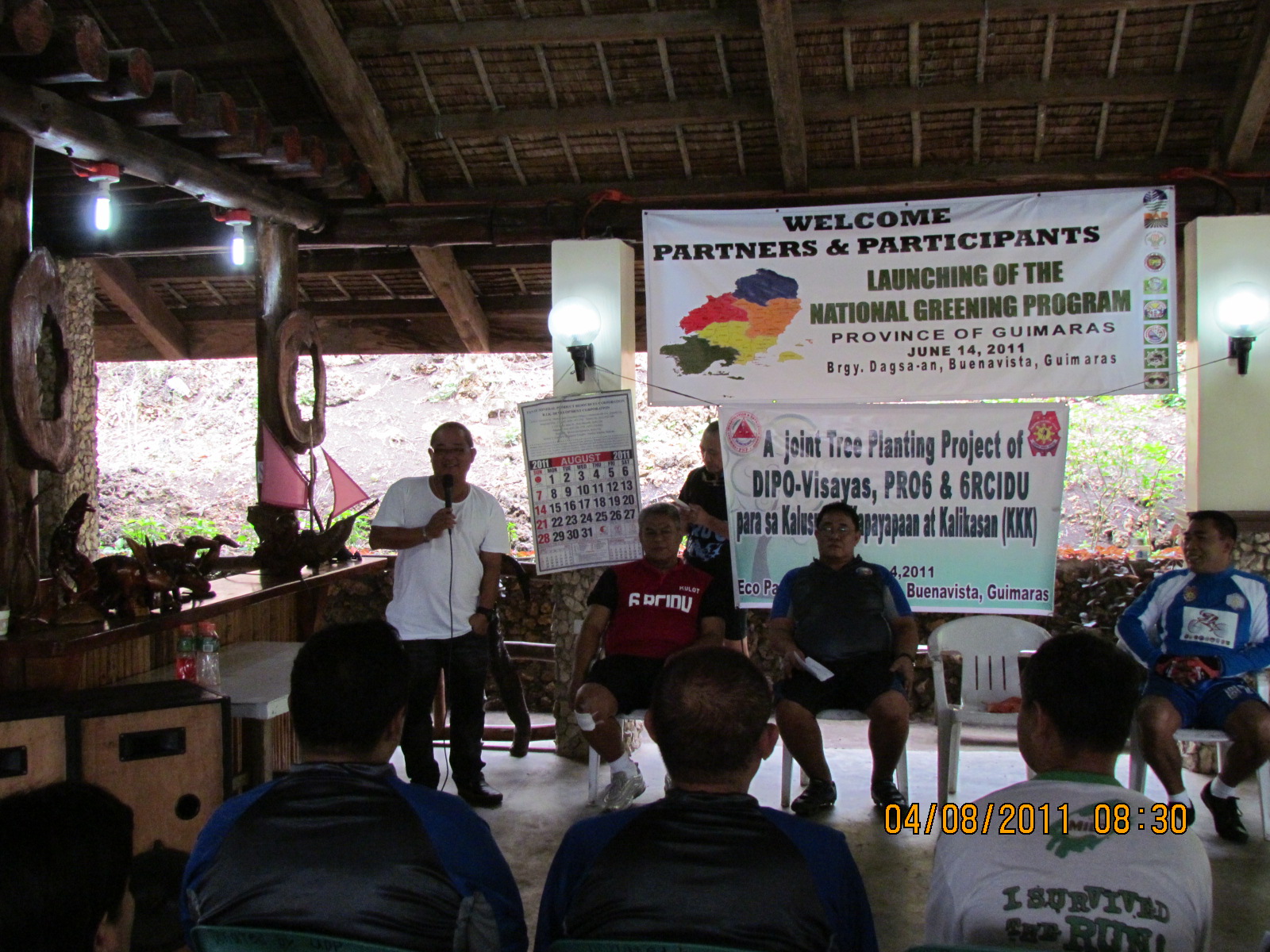The color photograph captures a lively scene of a National Greening Program event within a small pavilion featuring a wooden roof and open sides. The focal point is a man in a white T-shirt holding a microphone, presumably the speaker, standing to the left. To his right, several people are seated in green chairs, forming an attentive audience. Above them, prominently displayed, is a white banner that reads, "Welcome Partners and Participants, Launching of the National Greening Program, Province of Guimaras, June 14, 2011, Burgi, Dagestan, Buena Vista, Guimaras." A second banner below details, "A Joint Tree Planting Project of DIPO, Visayas, PR-06, and 6RCIDU, Paraca." The audience is actively listening to the presentation, focused on the launch of the program. Behind them, visible beyond the structure's open sides, is a rocky hillside dotted with vegetation, adding to the natural setting of the event. The overall atmosphere conveys unity and environmental commitment under the roofed, pavilion-like space on a significant occasion for community-driven environmental efforts.